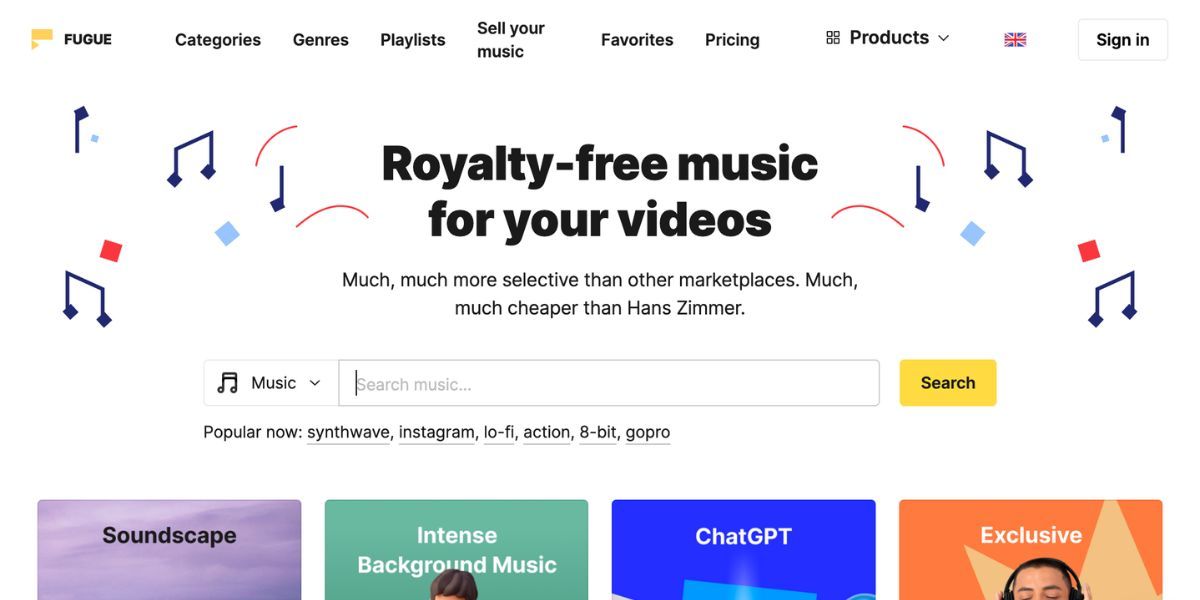Here is a detailed, cleaned-up caption:

---

This screenshot depicts a webpage focused on providing royalty-free music for videos. Located prominently in the center in bold black print is the phrase "royalty-free music for your videos," adorned with musical notes on either side. Directly beneath this, the text reads: "Much, much more selective than other marketplaces. Much, much cheaper than Hans Zimmer." Notably, the first "Much" and the "Much" starting the next sentence are both capitalized, as well as "Hans" and "Zimmer." Below this text, there is another musical note symbol, followed by the word "music" and a downward-facing arrow pointing to a search bar that reads "search music." Adjacent to the search bar on the right is a yellow button labeled "Search." Further down, four small rectangles appear: the first is purple and labeled "Soundscape"; the second is bluish and labeled "Intense Background Music."

---